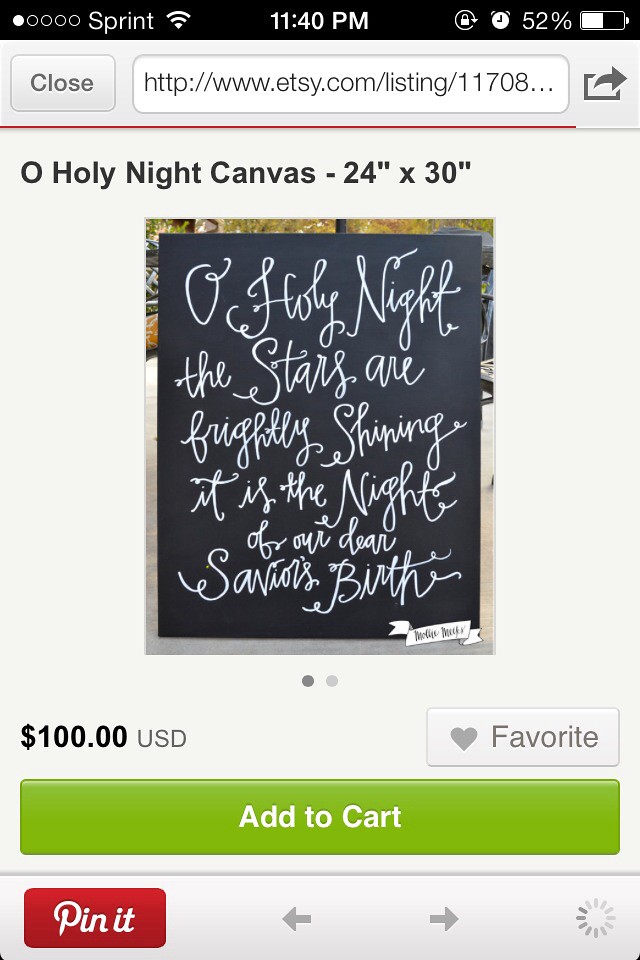This is a detailed screenshot from a mobile device, presumably a smartphone or tablet, connected to the Sprint network. It shows the time as 11:40 p.m. and the battery level is at 52%. At the top of the screen, icons for battery, alarm clock, Wi-Fi, and the Sprint signal strength are visible against a horizontal black bar, with white indicators and symbols, including the time display.

Beneath the black bar, there's a URL field displaying a web address from etsy.com against a white background. The page itself features a product listing for an item titled "O Holy Night Canvas," described in black letters as a 24 inch by 30 inch canvas. The canvas depicted in the middle of the screen has a black background with the words "O Holy Night" written in white cursive lettering, giving it a chalkboard effect.

The listing price for the canvas is $100, displayed below the product image in black text. At the bottom of the screen, a prominent green bar with "Add to Cart" written in white allows users to purchase the item. Adjacent to it is a red rectangle with the "Pin it" logo for Pinterest in white. There are also navigation and favorite buttons located below these elements, aiding further interactions with the product.